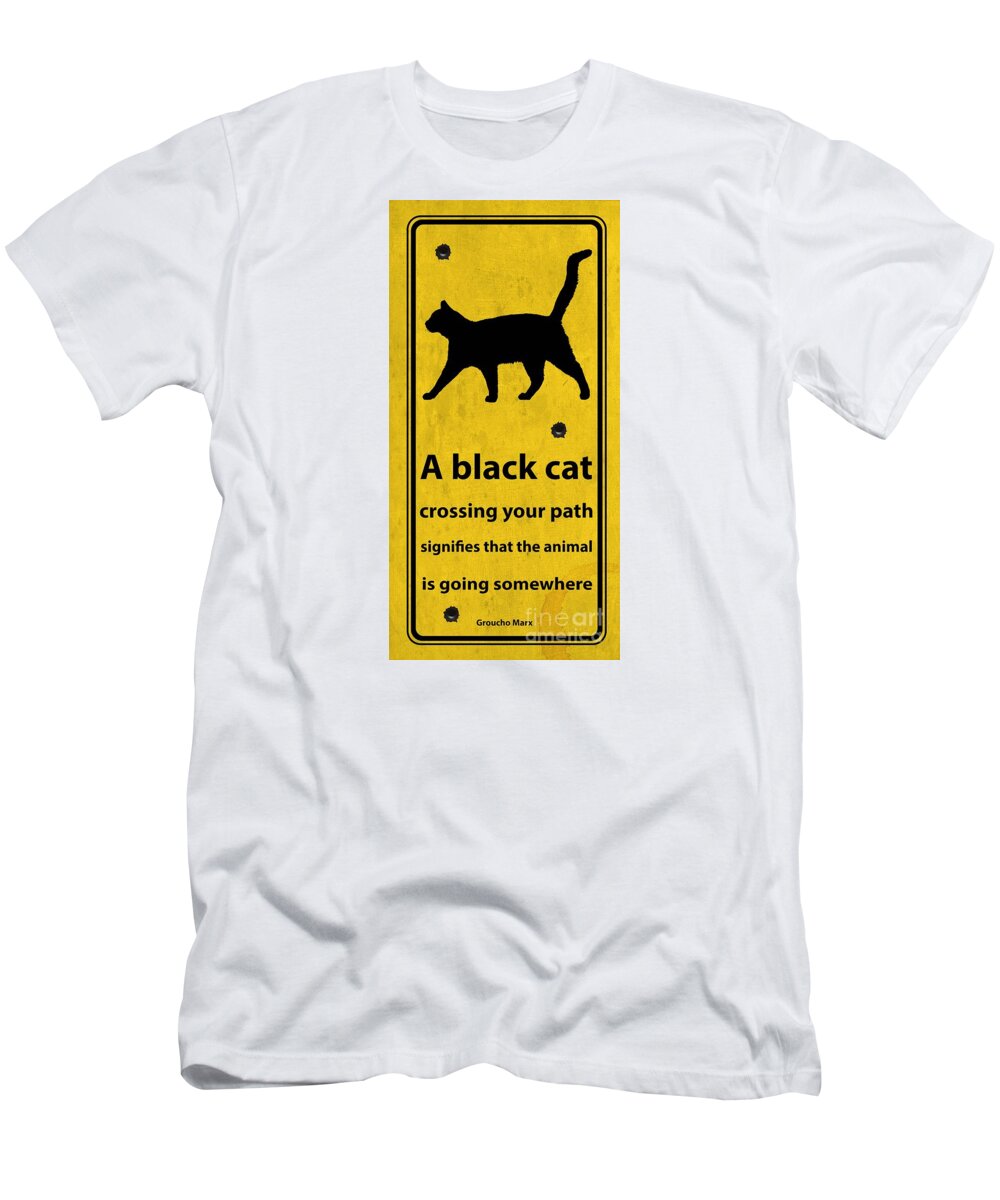This photograph showcases a white t-shirt laid flat on a white background, likely for advertisement or catalog purposes. The t-shirt features a prominent design: a long yellow rectangle extending vertically from the neck to the navel. Within this yellow rectangle is a striking silhouette of a black cat walking, accompanied by small paw prints in the top left and bottom right corners. The rectangle contains the witty text, "A black cat crossing your path signifies that the animal is going somewhere," suggesting a counter-narrative to superstitions about black cats. Below this main text is some smaller, difficult-to-read black writing, alongside a small black spot. Additionally, a faint watermark from Fine Art America is visible across the image, indicating it's likely for an art or merchandise platform.